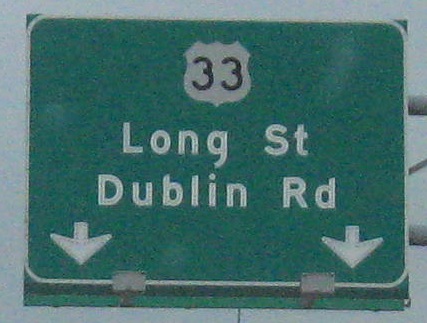This close-up image features a green highway sign in the shape of a square. The vibrant green background prominently displays the text "Long Street, Dublin Road" in bold white letters. At the bottom left and right corners of the sign, two white arrows point downward, indicating directions for motorists. Positioned at the top center of the sign is a white shield, emblazoned with the number "33" in black, signifying the highway or route number. The sign is secured to a sturdy pole with visible metal brackets. Additionally, there are two spotlights mounted beneath the sign, ensuring it is well-illuminated for nighttime visibility.